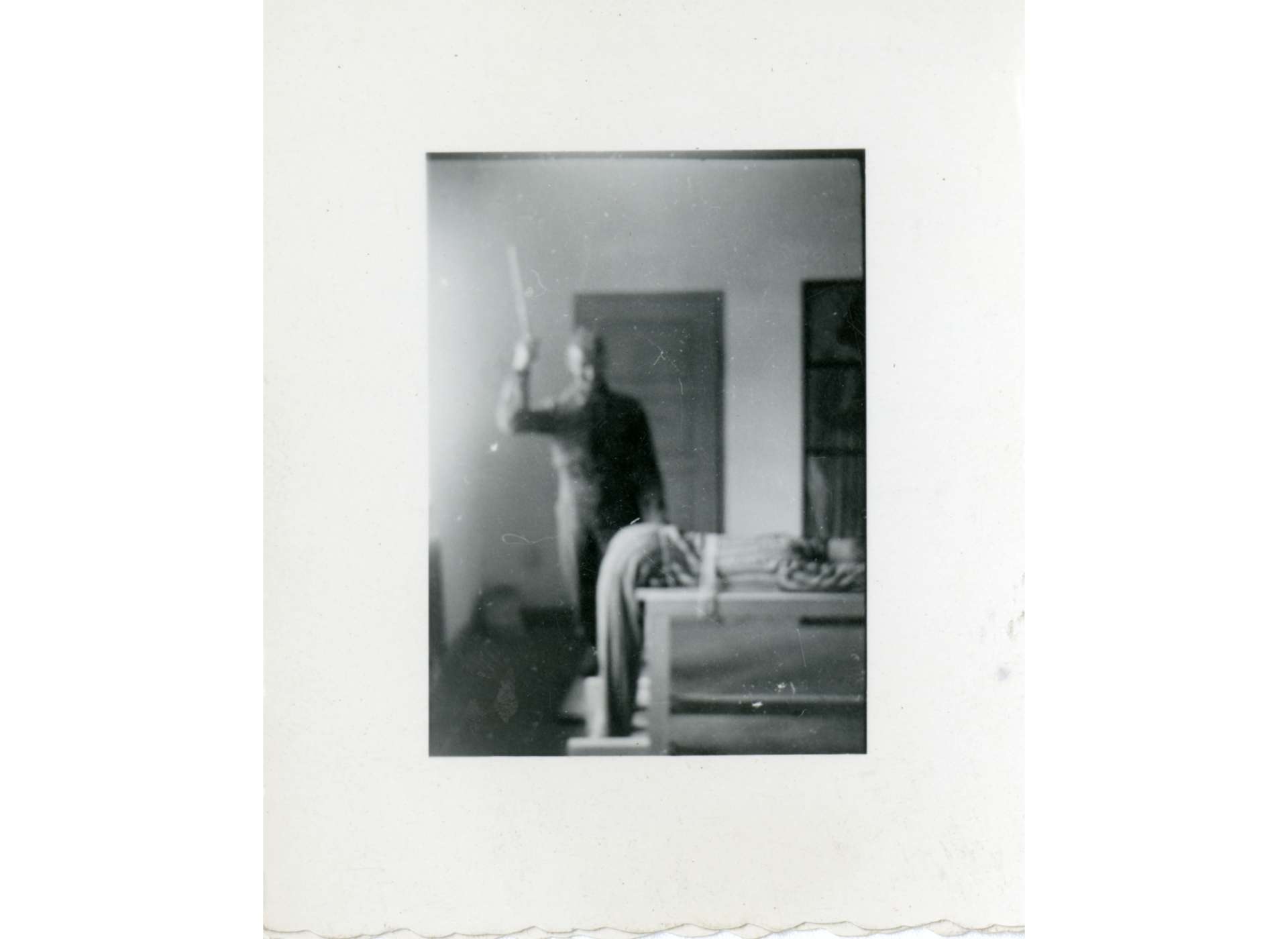This black and white photograph, which appears to be quite old and possibly from a book, shows a disturbing scene set in a small room. In the center of the image, a person is bent over a table or bed, seemingly strapped down with their hands positioned above their head, wearing pants and a long-sleeved shirt. Standing behind the strapped-down individual is a man, possibly wearing a long-sleeved jumpsuit or uniform, raising a stick or baton as if preparing to strike the person on the buttocks. The room features a couple of doors in the background and possibly a window or room separator to the right. The photograph includes a weathered edge at the bottom, adding to its antique appearance.